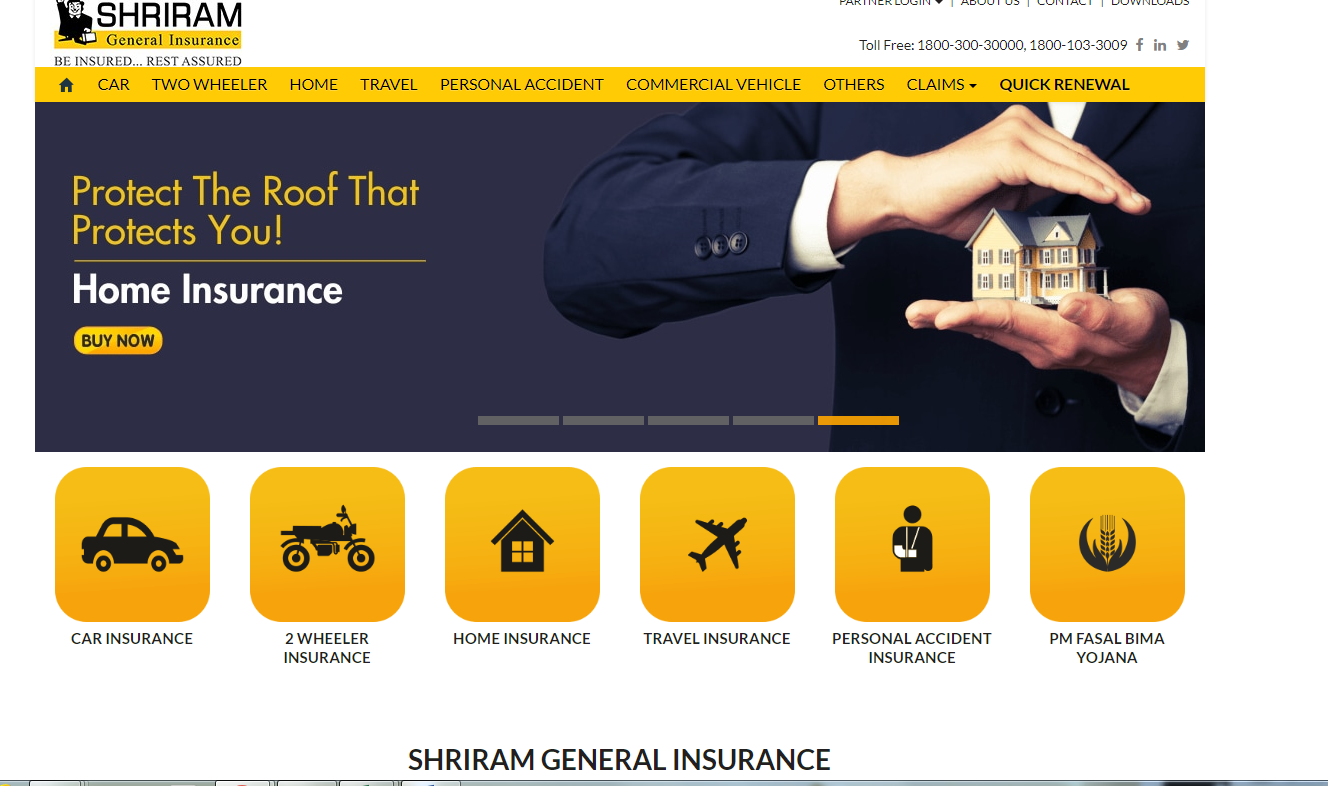The image is a promotional graphic for Shriram General Insurance, featuring a variety of elements and details. At the top, the text "Shriram General Insurance" is prominently displayed within a yellow bar. To the left of this text, there is a cartoon character illustration of a man dressed in a black suit. In the upper right corner, the options "Partner Login," "About Us," "Contact," and "Download" are listed, with a toll-free number situated underneath these options.

On the left-hand side, the slogan "Be Insured, Rest Assured" is featured. Below this, another yellow section includes various insurance categories with icons next to each label: "Car," "Two-Wheeler," "Home," "Travel," "Personal Accident," "Commercial Vehicle," "Others," "Claims," and "Quick Renewal."

Further down, the image depicts a man in a suit with only his hands visible. His hands are cupping a small yellow house with a gray roof. Adjacent to this visual, the text reads "Protect the Roof that Protects You," with "Home Insurance" written in white text beneath it and a small yellow "Buy Now" button nearby.

The lower portion of the graphic contains multiple yellow boxes labeled "Car Insurance," "Two-Wheeler," "Home Insurance," "Travel Insurance," "Personal Accident Insurance," and "PM Faisal Bima Yojana," each accompanied by corresponding icons. The graphic closes with the company name "Shriram General Insurance" once again at the bottom.